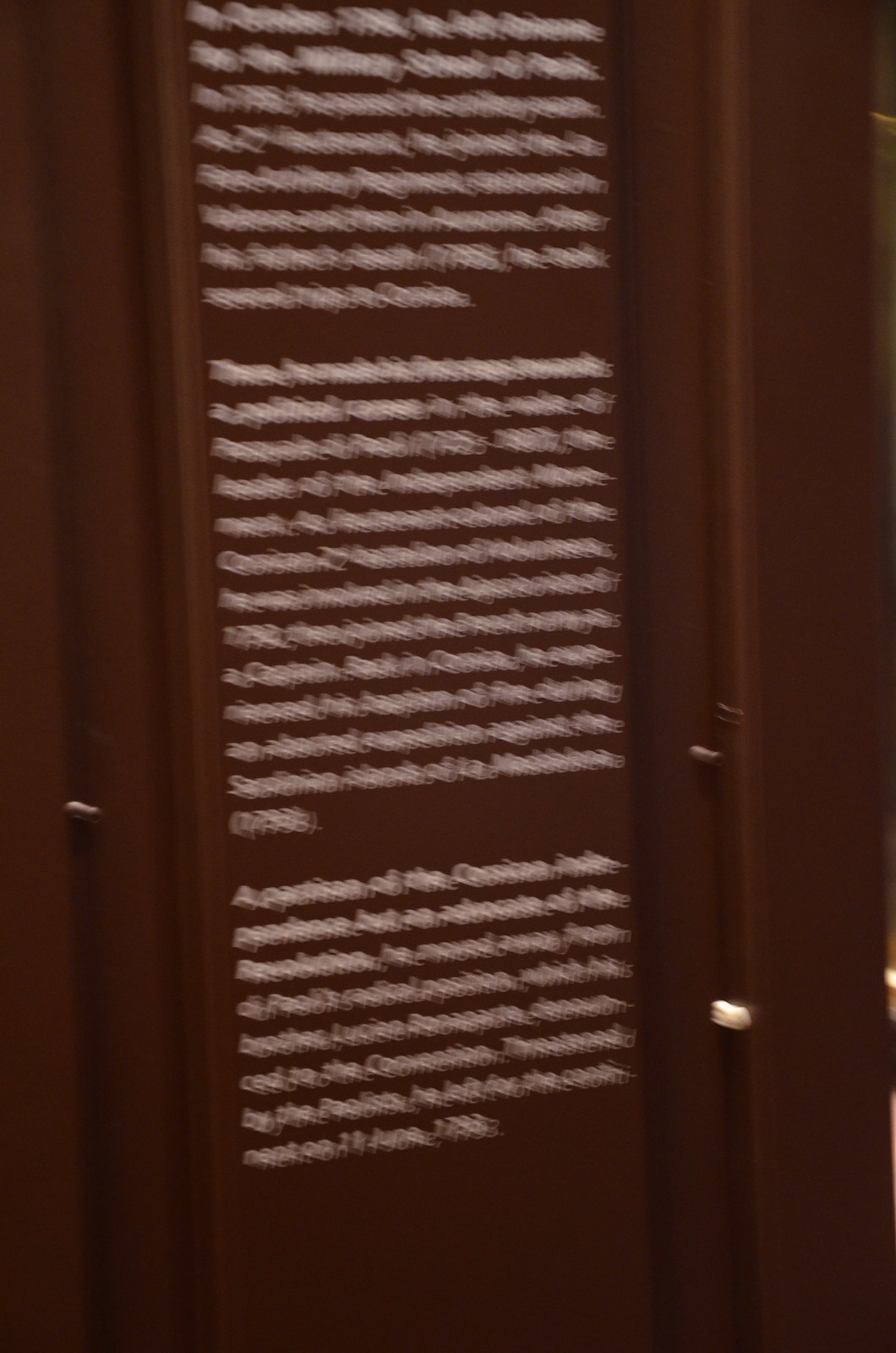This is a very low-quality and blurry photograph of a wall or a door that appears to be made of dark brown wood. Scattered across the surface is what looks like a mounted plaque of the same brown wood color, blending seamlessly with the background. The plaque contains three paragraphs of white, clearly visible text, though the blurriness makes reading the text difficult. The writing seems to describe a historical figure involved in a political career and the Corsican independence movement. Snippets of the text include phrases like "a political career," "a partisan of the Corsica," "revolution," and "21 June 1793." There is what appears to be a chrome door handle in the lower right part of the photograph, indicating that the plaque might be on an actual door. The context and structure of the text suggest it is a detailed informational description typical of what one might find next to an exhibit in a museum.